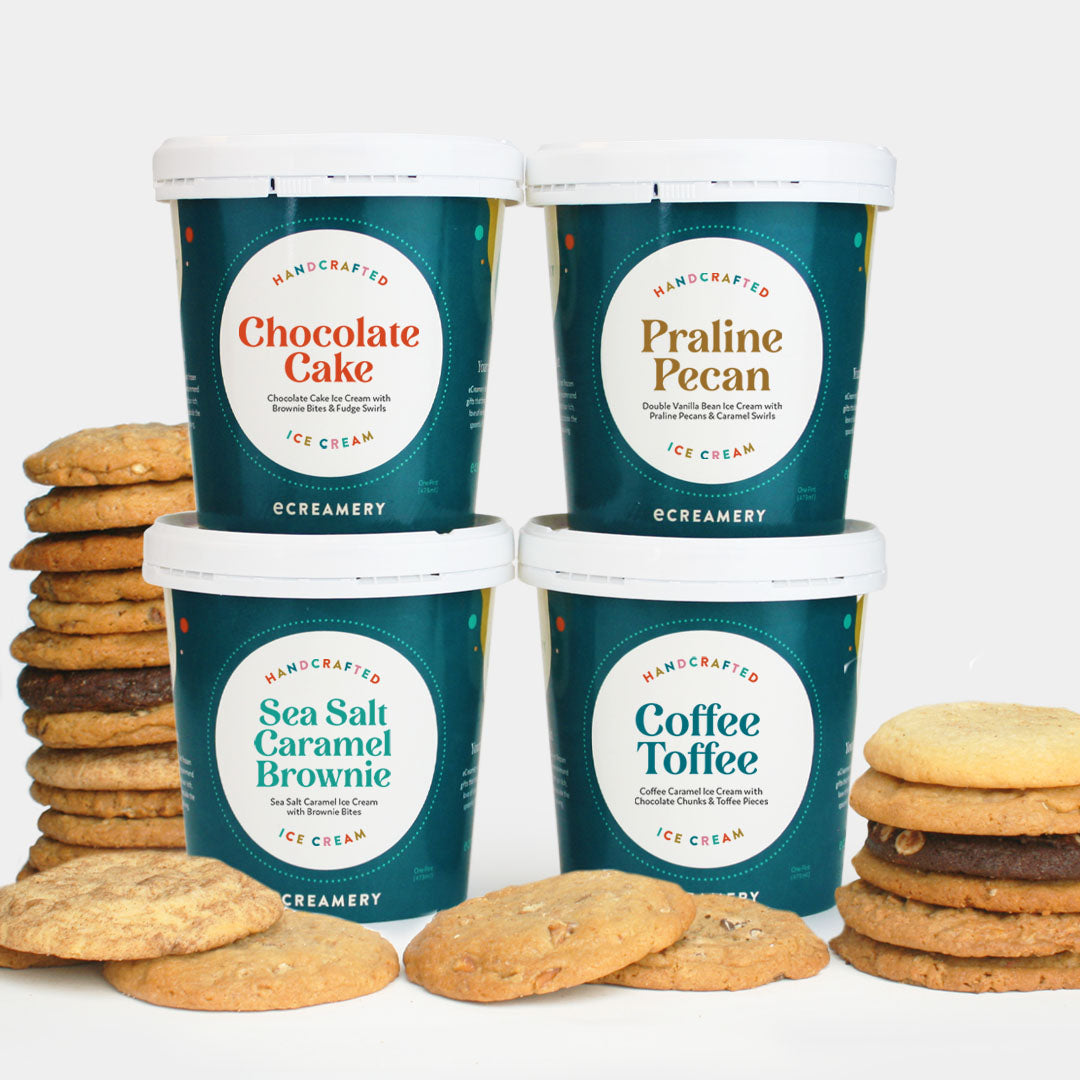The product marketing image showcases four pint containers of handcrafted E Creamery ice cream varieties, each adorned with distinct color-coded labels on a dark blue-green background. The flavors are Chocolate Cake with brownie bits and fudge swirls, Praline Pecan with double vanilla bean ice cream, caramel swirls, and praline pecans, Sea Salt Caramel Brownie with sea salt caramel ice cream and brownie bites, and Coffee Toffee with coffee caramel ice cream, chocolate chunks and toffee pieces. These pints are arranged in a stack at the center, with two on the bottom and two on top. Surrounding the ice cream containers are stacks of flat, round cookies in light tan, gold, and dark brown hues. The cookies are positioned in front, behind, and beside the pints, creating an inviting, artisanal display against a plain white background, highlighting the handcrafted nature of the treats.